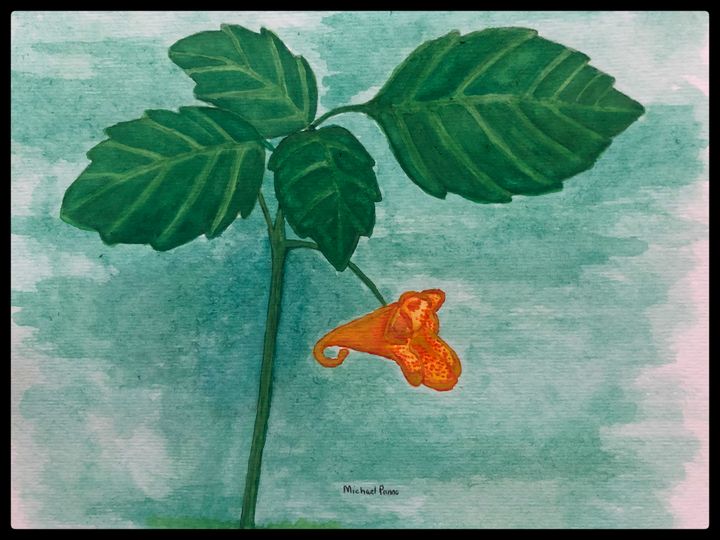This image is a semi-realistic painting by Michael Pena. The artwork appears to be a multimedia piece, primarily utilizing watercolor. It depicts a plant with a single budding flower. The plant features a central stem from which four deep green leaves with lighter green veining extend in different directions. Below the leaves, a smaller stem supports a flower bud that is predominantly orange with hints of red and shades of peach, adorned with small red dots. The background transitions from a greenish-blue or turquoise hue to a muted white, giving a blurred, soft-focus effect. The artist's name, Michael Pena, is subtly signed at the bottom in small black letters.